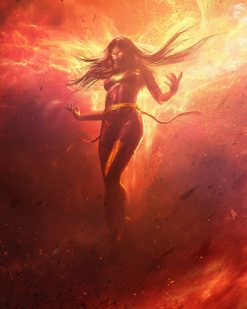This is an intricately detailed fantasy-themed poster of a superhero-like woman with long, dark, flowing hair, rising majestically from a swirling inferno of flames. Her eyes glow with an intense orange-yellow light, suggesting her potent ability to command fire. She is dressed in a skin-tight, deep red jumpsuit paired with striking thigh-high yellow or golden boots. A flowing yellow sash, wrapping her waist, trails behind her, adding dynamic movement to the scene.

The background is a tempest of dark reds and fiery oranges, with flames encircling and engulfing the figure, making it appear as if she is emerging from the heart of a blaze. Her hair, infused with fire, streams around her, enhancing the sense of power and motion. She stands confidently, her left leg straight and her right leg slightly bent, as if poised to summon or control the fire around her. Both hands are outstretched beside her, palms open, giving the impression that she is about to unleash a formidable force.

The overall composition, with its vivid, fiery colors and dramatic pose, suggests a powerful, otherworldly being, reminiscent of characters found in comic books like those from Marvel or DC. The absence of text allows the striking visuals to tell the story, with the glowing, flame-clad figure dominating the center of the image, her feet barely visible amidst the encircling flames and the light emanating from behind her.